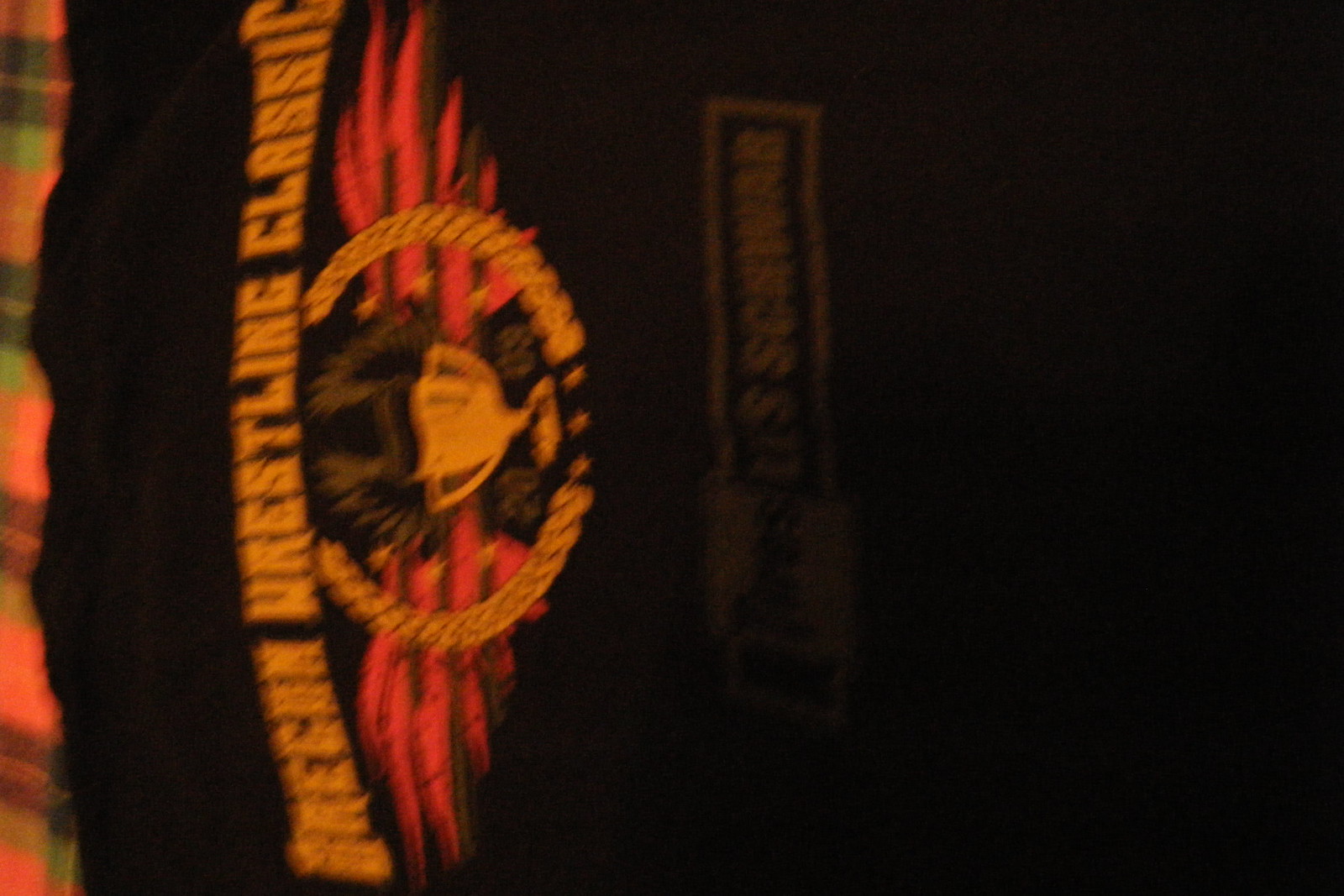The image is very blurry, with a majority of the right side being completely black. On the left side, the image appears to be slightly tilted. After closer inspection, it seems to depict a black T-shirt bearing the inscription "Oregon Wrestling Classic" in gold lettering. The central design features a gold trophy with handles, encircled by an arrangement resembling wheat, also in a rounded shape. Behind the trophy, red flames add a dynamic backdrop, while the area above the trophy shows black feathers with gold outlines, although the details are indistinct. The background to the left of the T-shirt includes a fuzzy plaid pattern. Below the trophy, there is a faintly visible box with some difficult-to-read lettering that includes "SC" and vaguely resembles scissors, although the exact details remain unclear due to the poor image quality.